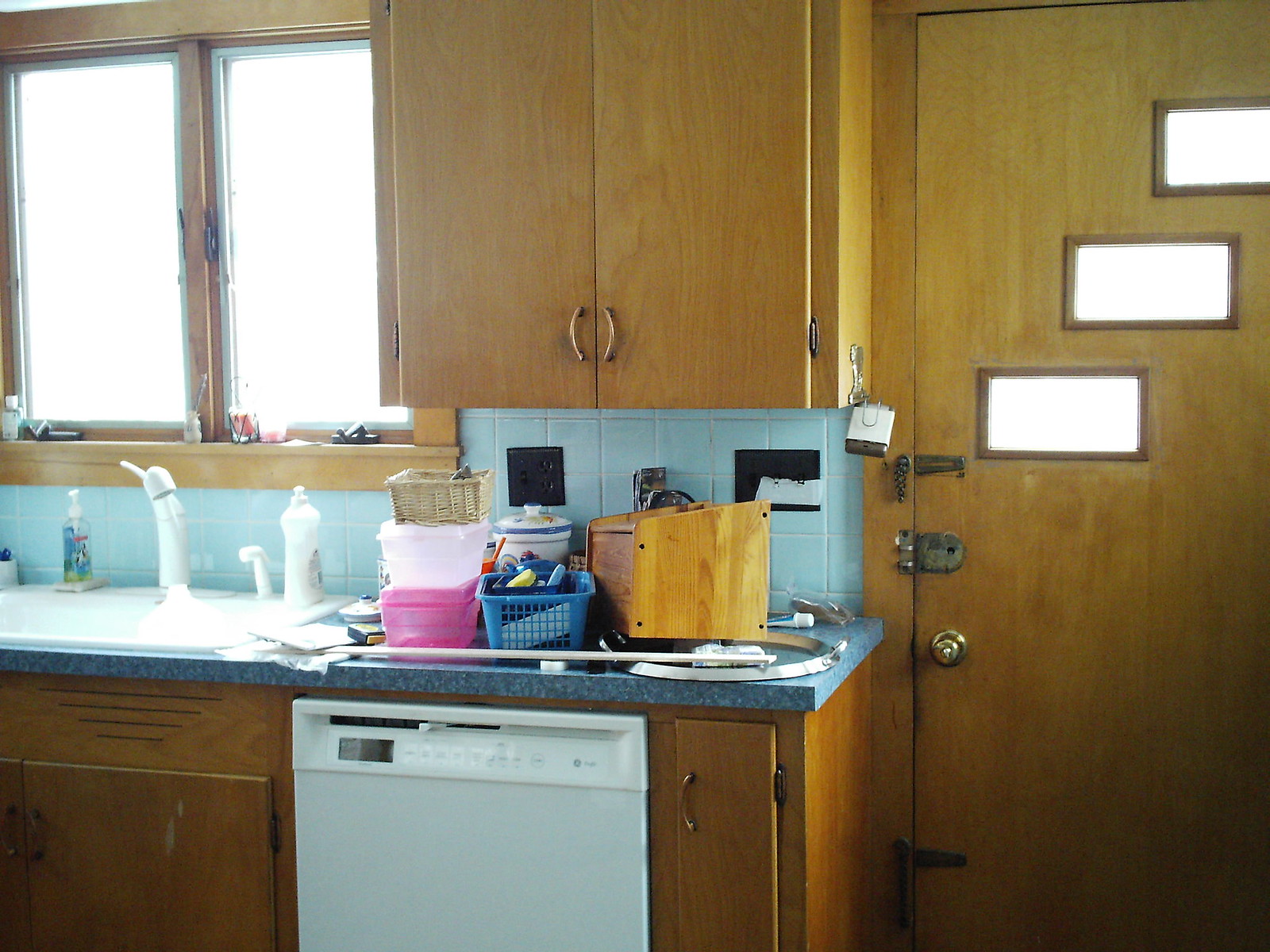This photograph showcases the interior of an old-fashioned kitchen, characterized by its distinctly 1970s aesthetic. The space is defined by medium brown wooden cabinets, creating a warm, retro atmosphere. The kitchen features a baby blue tile backsplash, adding a vintage touch to the overall design. 

On the right side of the image, there is an exterior door made of the same brown wood with a doorknob, a deadbolt above it, and a latch lock. This door is distinguished by three horizontal rectangular windows arranged diagonally from the lower left to the upper right. Adjacent to the door, an upper cabinet with curved handles in the same brown wood hangs above a blue countertop. Below the countertop, a white sink is paired with a white dishwasher, flanked by lower cabinets matching the upper ones.

In the top left corner, a window split into two sections (left and right) with a brown wooden frame allows natural light to enter the room. The countertop beneath this window is cluttered with various items, including a brown wooden bread box, a small blue basket holding miscellaneous objects, a pink Tupperware container with a white Tupperware container stacked on top, and a very small wicker basket perched on the topmost container. There seems to be a glass and metal pot lid placed underneath the bread box. The kitchen also features black outlets and switch plates embedded within the blue tiled backsplash, adding to the functional yet nostalgic ambiance of the space.